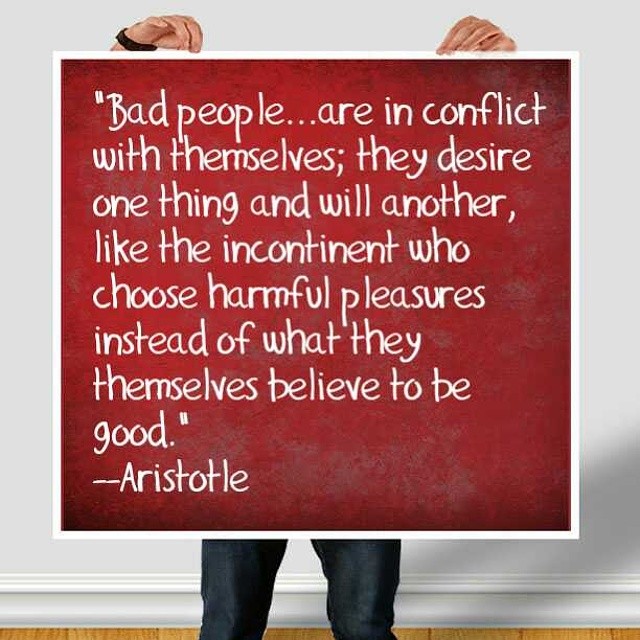A square image features a partial view of a person standing against a white wall with a light brown wooden floor at the bottom edge. The main focus is a red sign with a white border and white handwritten-style text, held by two hands at the top and displaying two upper legs clad in jeans at the bottom. The sign, slightly textured with gray splotches, bears the quote: "Bad people are in conflict with themselves. They desire one thing and will another, like the incontinent who choose harmful pleasures instead of what they themselves believe to be good. - Aristotle."